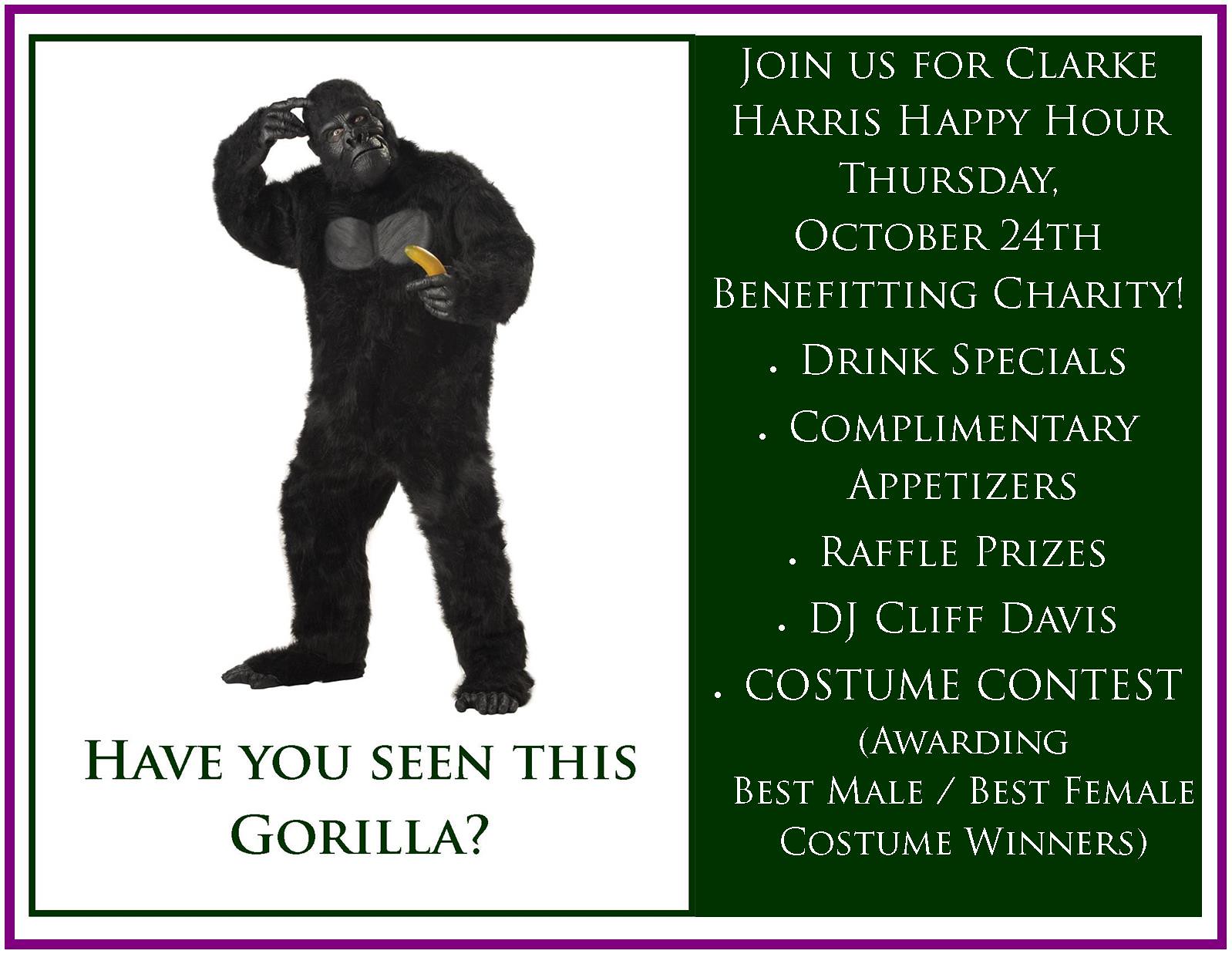The promotional poster is divided into two distinct sections with a purple outer border and a green inner border. The left two-thirds feature a white background with the image of a man in a gorilla suit holding a banana in his left hand and scratching his head with the other. Underneath the image, in dark green capital letters, it reads, "Have you seen this gorilla?" The right one-third has a dark green background with white text that invites viewers to "Join us for Clark Harris Happy Hour" on Thursday, October 24th. This section provides details about the event, including its charitable cause, drink specials, complimentary appetizers, raffle prizes, a DJ performance by Cliff Davis, and a costume contest with awards for Best Male and Best Female costumes.